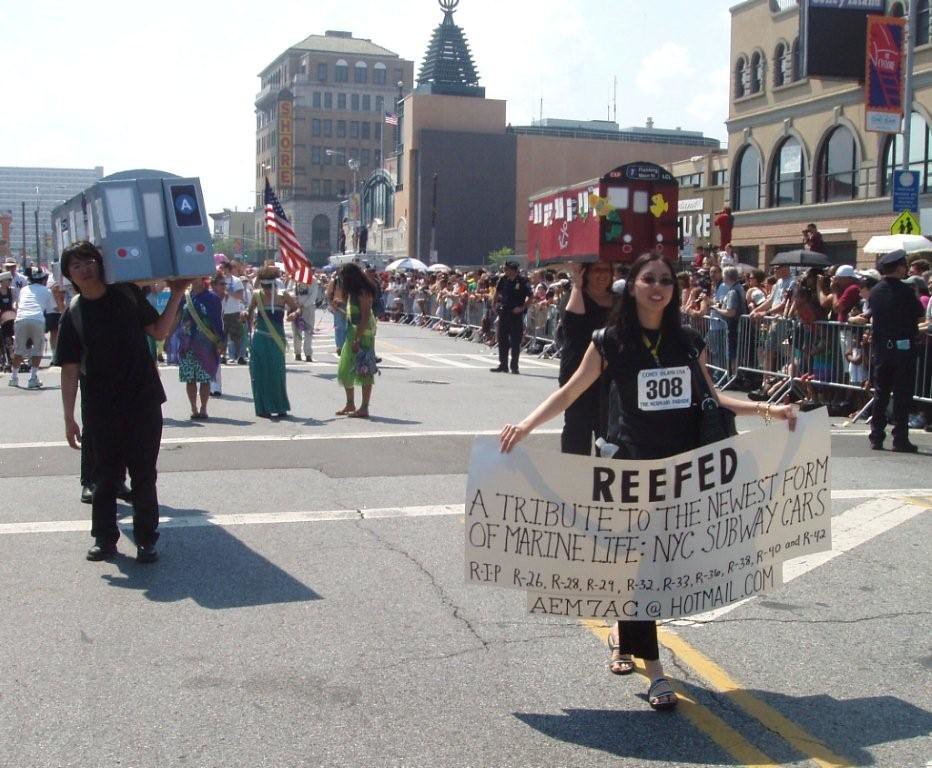This photo captures a vibrant daytime parade in a small city, featuring a significant mix of events, tributes, and cultural elements. At the forefront, on the right side, is a woman with long dark hair, wearing sunglasses and a black shirt adorned with a tag numbered 308. She grasps a large white sign that reads, "REEFED, a tribute to the newest form of marine life, NYC subway cars. RIP R26, R28, R29, R32, R33, R36, R38, R40, and R42," with a contact email, AEM7AC at Hotmail.com. Close by, two individuals are holding up a model of a subway car display. In the background, a group of people dressed in traditional Polynesian or Hawaiian attire, featuring green and purple dresses, march along the parade route. The street is lined with spectators behind bike fencing and barriers, some using umbrellas for shade, with police officers maintaining order. The setting is characterized by nearby city buildings, adding to the lively urban atmosphere.